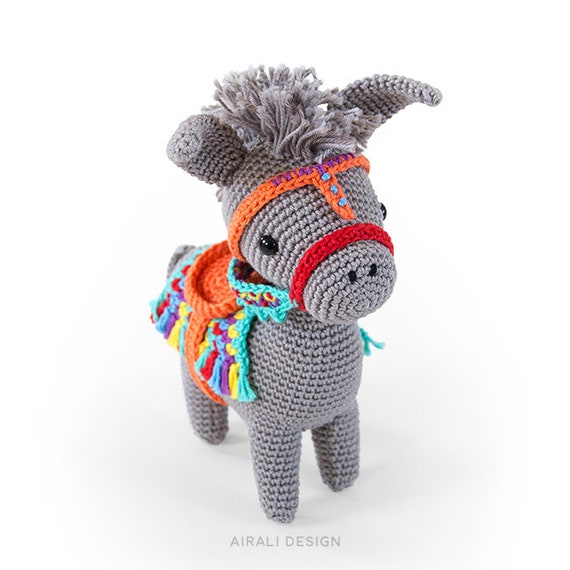The image features a detailed close-up of a grey crocheted donkey toy, designed to capture the eye with its charming and expressive features. The donkey's pointed ears stand upright, and it sports a tuft of grey yarn resembling a mohawk atop its head. A black beard complements its expressive eyes, enhancing its character. This toy is adorned with a colorful saddle blanket that showcases intricate patterns in bright hues such as orange, blue, green, yellow, and purple, all fringed with tassels. The saddle itself is primarily orange and is held in place by vivid red straps that go over the donkey's head and under its chin. The clean, white background of the image ensures that the crocheted toy remains the main focal point. At the bottom of the image, the text "Airali Design" is clearly visible, adding a professional touch to the playful scene.